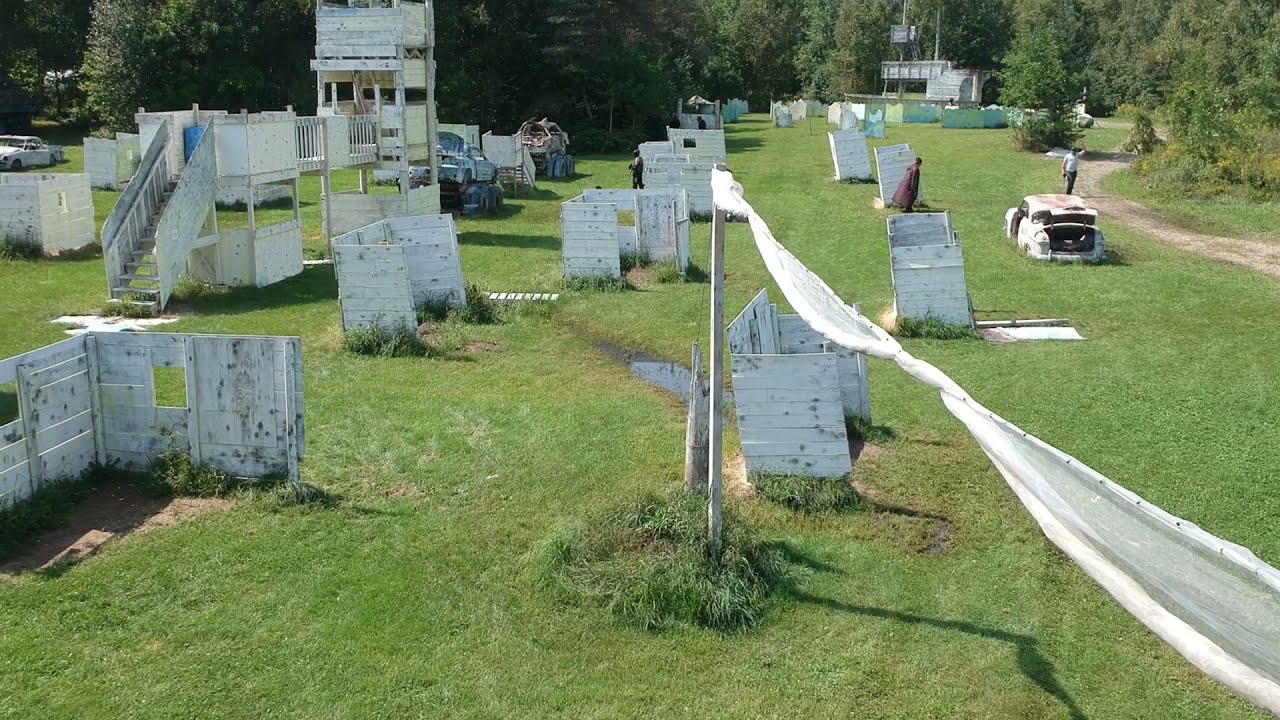The image captures an odd, horizontally rectangular field with lush green grass and several dilapidated, partial wooden structures scattered about. These structures resemble two- and three-sided weathered white walls, speckled with black and brown moldy spots, and appear like old, broken-down shed parts and fences. Towards the left, an intricate arrangement of these wooden structures features stairs leading up to a platform, connected by a small bridge to a taller section. The entire scene is shot from a slightly elevated angle, providing a comprehensive view of the area.

In the background, you can see dense trees spanning from the right to the left, and a dirt path curving through the upper right corner of the image. Several people are visible, walking among the peculiar wooden formations. The sun is shining, although the sky isn't visible. To the right of the scene, an old, wheel-less, white car rests abandoned on the grass near the dirt path, while more similarly derelict cars are seen off to the left. The overall ambiance suggests a sunny, deserted site with no text or signs in view, leaving the decrepit constructs and scattered vehicles starkly exposed amidst the greenery.